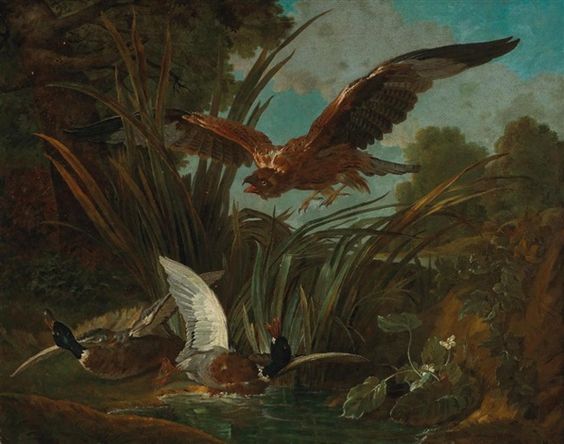In this detailed painting, we see an intense moment in nature captured with striking realism. The scene depicts two mallard ducks in a murky lily pond, their wings splayed in a frantic attempt to escape a menacing bird of prey descending from above, possibly a vulture or falcon. The predator, with talons extended and beak open, casts an ominous shadow over the ducks.

The overall palette of the painting is dominated by dark, earthy tones—greens, browns, and dirty blues—reflecting a gloomy, dim day. The pond is partially obscured by reeds and dotted with lily pads, one of which features delicate flowers to the right. Grass emerges sporadically from the murky water, adding to the sense of a marshy environment.

In the background, a large green tree occupies the left side, while the right side reveals a brown, hill-like formation leading into the water. The sky is overcast with dirty blue clouds, enhancing the foreboding atmosphere. Skillfully rendered without visible brush strokes, the painting immerses the viewer in a meticulous, yet almost haunting, depiction of wildlife.